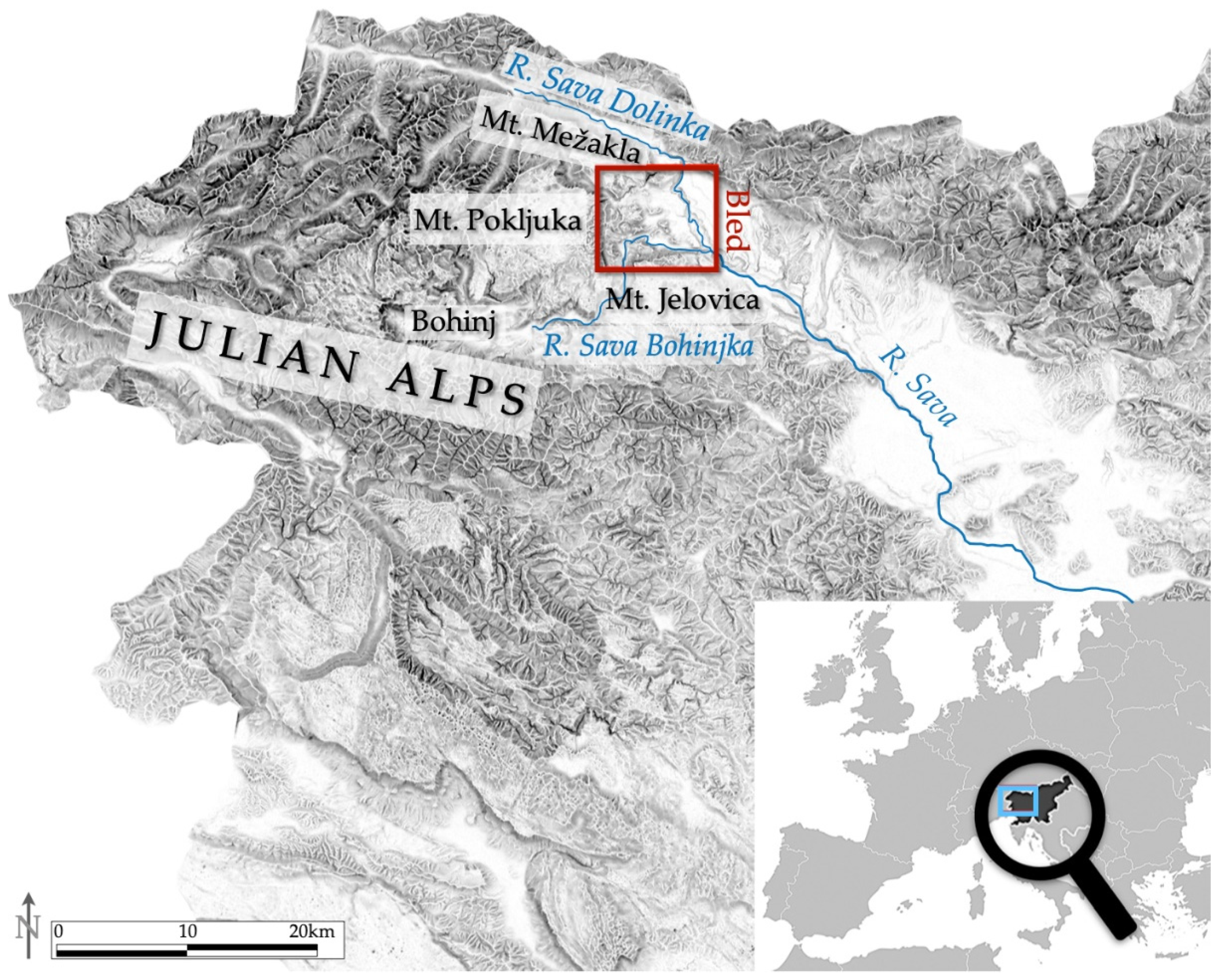The black and white image depicts a detailed map of the Julian Alps. Prominently, there is a white rectangle labeling the Julian Alps in the upper left corner. Several significant locations are marked in different colors: Bled is highlighted in red with a square around it, while the Arsava river and Bohinga, Arsava Dolinka, and Arsava Bohinga locations are marked in blue. Other points of interest include Mount Tujuca, Mount Jolovica, Mount Mzakhla, and Mount Poklodjika labeled in black. There is a compass in the bottom left corner indicating the north direction, accompanied by a bar for measuring distances in kilometers up to 20 km. The bottom right corner features a zoomed-out section of the map, with a magnifying glass effect highlighting the specified area in focus.